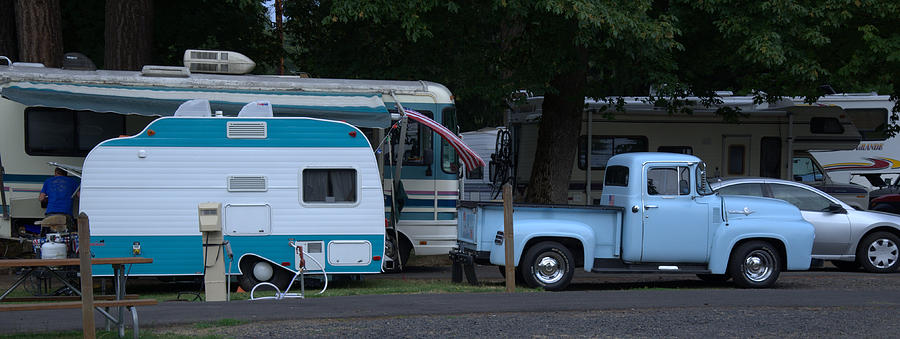In this detailed photograph of a campground, multiple vintage and modern vehicles are scattered across the scene, creating a nostalgic yet lively atmosphere. The main focus is a charming vintage camper from the 1950s, which is painted in an aqua and white scheme. It’s attached to a vintage truck from the same era, clad in a contrasting robin's egg blue, adorned with chrome detailing. The photograph captures this endearing setup parked on a gray paved area, with a patch of green grass and a picnic table in the foreground, hinting at a cozy campsite scene.

The background is filled with an array of RVs; to the left, a modern silver sedan can be seen parked next to a Winnebago-style C-Class RV and a fifth wheel trailer further back. An imposing A-Class RV with an extended sunshade also features prominently. The vintage blue truck and camper duo is juxtaposed against these modern counterparts, adding charm to the setting.

Although the sky is barely visible, just a sliver of it peeking through in the left background, the periphery of the image reveals a dense backdrop of tree trunks and lush green foliage, suggesting the campground is nestled within a verdant, forested area. The overall ambiance hints at a serene, perhaps late-afternoon setting, with softened shadows indicating the sun is approaching the horizon, casting a tranquil light over the scene.